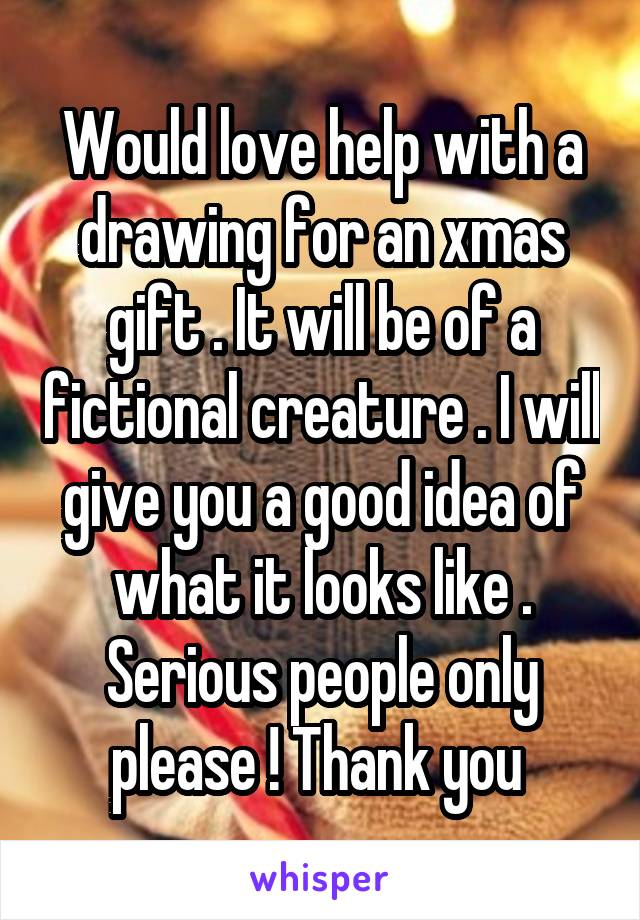The image features a white coffee mug with a dark blue, geometrical crocheted pattern on the outside, holding a red and white candy cane hooked over the lip. The mug rests on a tan or beige cloth, placed against a blurry, golden-tan background that hints at out-of-focus lights. Overlaying the entire picture is a prominent block of white text with a black outline, which reads: "Would love help with a drawing for a Christmas gift. It will be of a fictional creature, I will give you a good idea of what it looks like. Serious people only, please, thank you." Below this text, within a thin, gray-outlined white rectangle, the word "whisper" is displayed in purple lowercase letters.